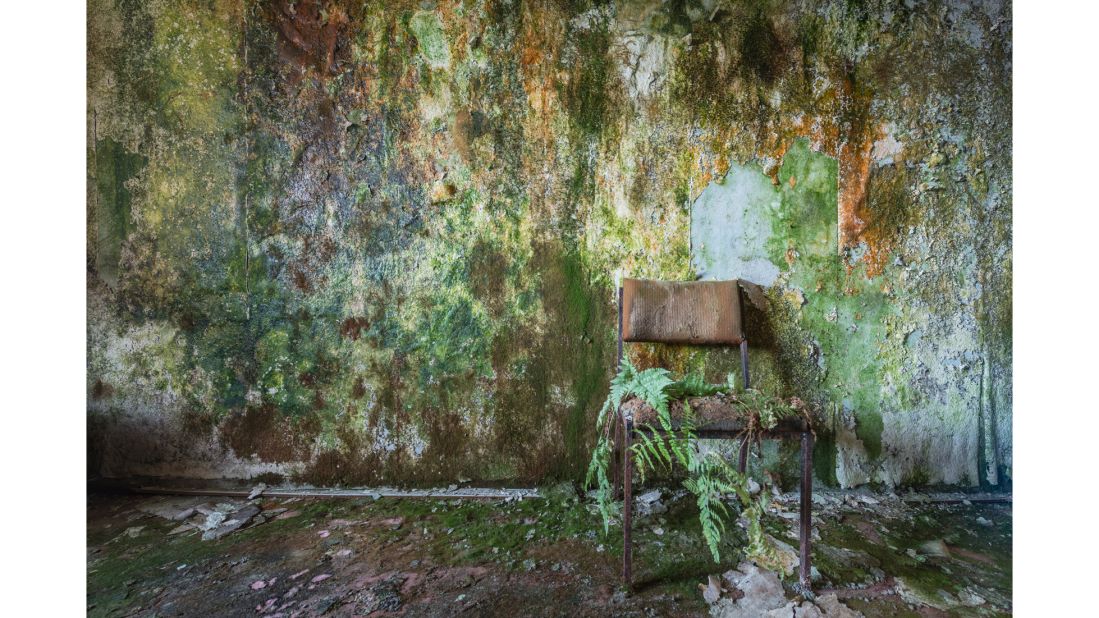The image showcases a highly dilapidated and decaying room, clearly abandoned for a long time. Dominating the scene is a wall meeting the floor, both covered in a patchy mix of green moss, algae, mold, and rust, creating a vibrant and grimy texture. The floor is littered with paint and wall chips, adding to the overall state of decay. Central to the right is an extremely weathered brown metal chair, draped in overgrown fern-like plants. The chair, resembling those found in waiting rooms, is partially submerged in the rampant moss and appears damp and worn. The overall atmosphere of the room suggests a post-apocalyptic or long-neglected environment, with a photorealistic quality that highlights every grimy detail.